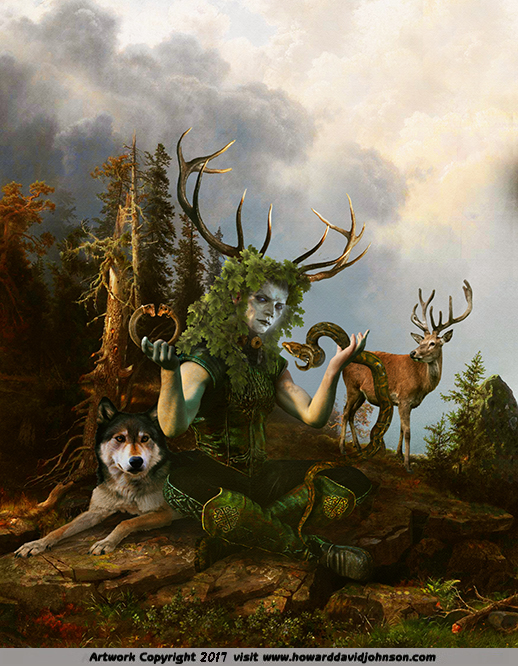This fantasy-themed AI artwork features a central figure sitting cross-legged on a mountaintop, presenting a blend of human and nature elements. The person has a face painted completely white and deer antlers emerging from their head, which appears to be surrounded by a bed of leaves, giving the impression that their head is part tree. They are dressed in a dark green and black outfit, including a green leather vest, bare arms, black pants with a white pattern down the side, and green and gold leather boots. In their right hand, they hold a horseshoe, while their left hand raises a snake. Seated beside them is a husky dog, accentuating the woodland setting. The background reveals a mix of tall, dead pine trees and a standing deer with antlers, all under a sky transitioning to gray clouds. The bottom of the image displays the text "artwork copyright 2017," directing to www.howarddavidjohnson.com.